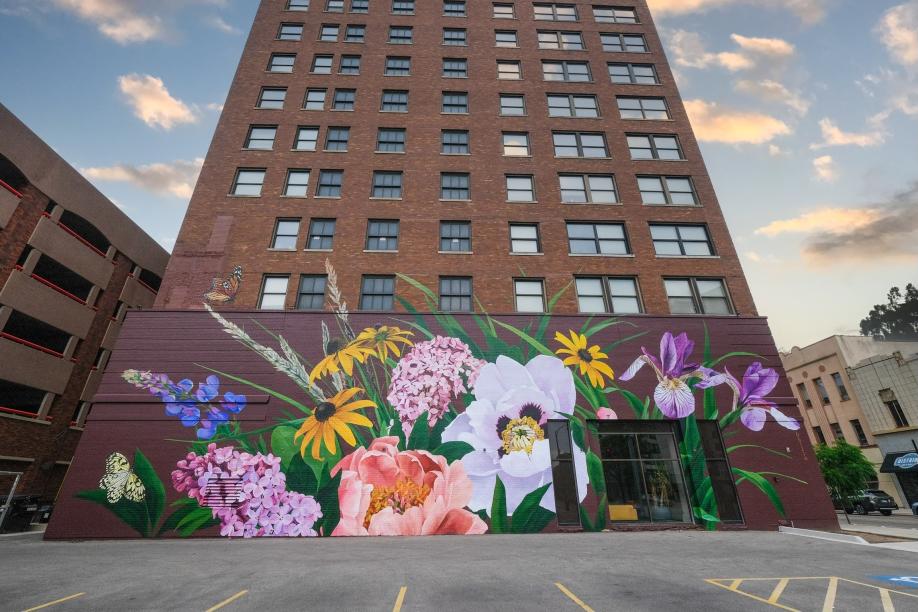The image depicts a tall brick building, estimated to be between eight to ten stories high, featuring numerous small windows that suggest it might be an apartment building. The first two stories are made of dark brown, reddish brick, transitioning to a lighter brown hue for the upper floors. On the right side of the building, there is a glass double door entrance, adjacent to a parking lot lined with yellow borders marking each parking spot.

A striking element of the image is a large, beautiful mural adorning the lower portion of the building's facade, primarily towards the left side and extending over the doorway. The mural, set against a black background, vividly portrays a variety of flowers. Prominent in the artwork are black-eyed Susans with their yellow petals and black centers, bluebells, purple irises, lilac flowers, and white lilies. Light purple and pink flowers also contribute to the garden-like scene, creating a vibrant and colorful display that enhances the building's exterior. Additionally, to the left of the main building, a beige parking garage with open windows is visible, made from beige concrete, further contextualizing the urban environment.